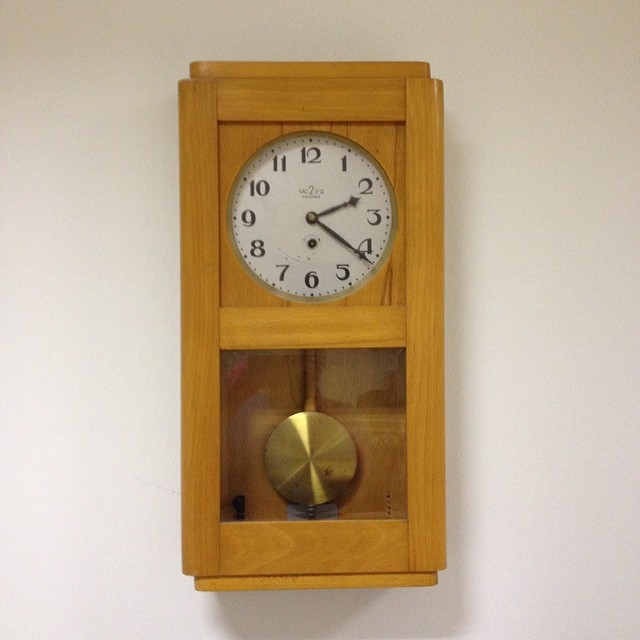This photograph showcases a high-quality image of a vintage wall clock with an intricate design. The clock features a blondie-yellow wooden frame, prominently displaying the natural wood grain. At the top, the round white clock face is adorned with bold black numbers and sleek black hands, providing a classic look. Below the clock face, a gold pendulum is visible through a glass covering, which reflects subtle light and shadows. Inside the glass enclosure, a small gray object is noticeable beneath the pendulum, and a tiny black metal piece is positioned to one side. The clock is mounted on a clean, white wall, adding contrast and highlighting the elegant details of the timepiece.